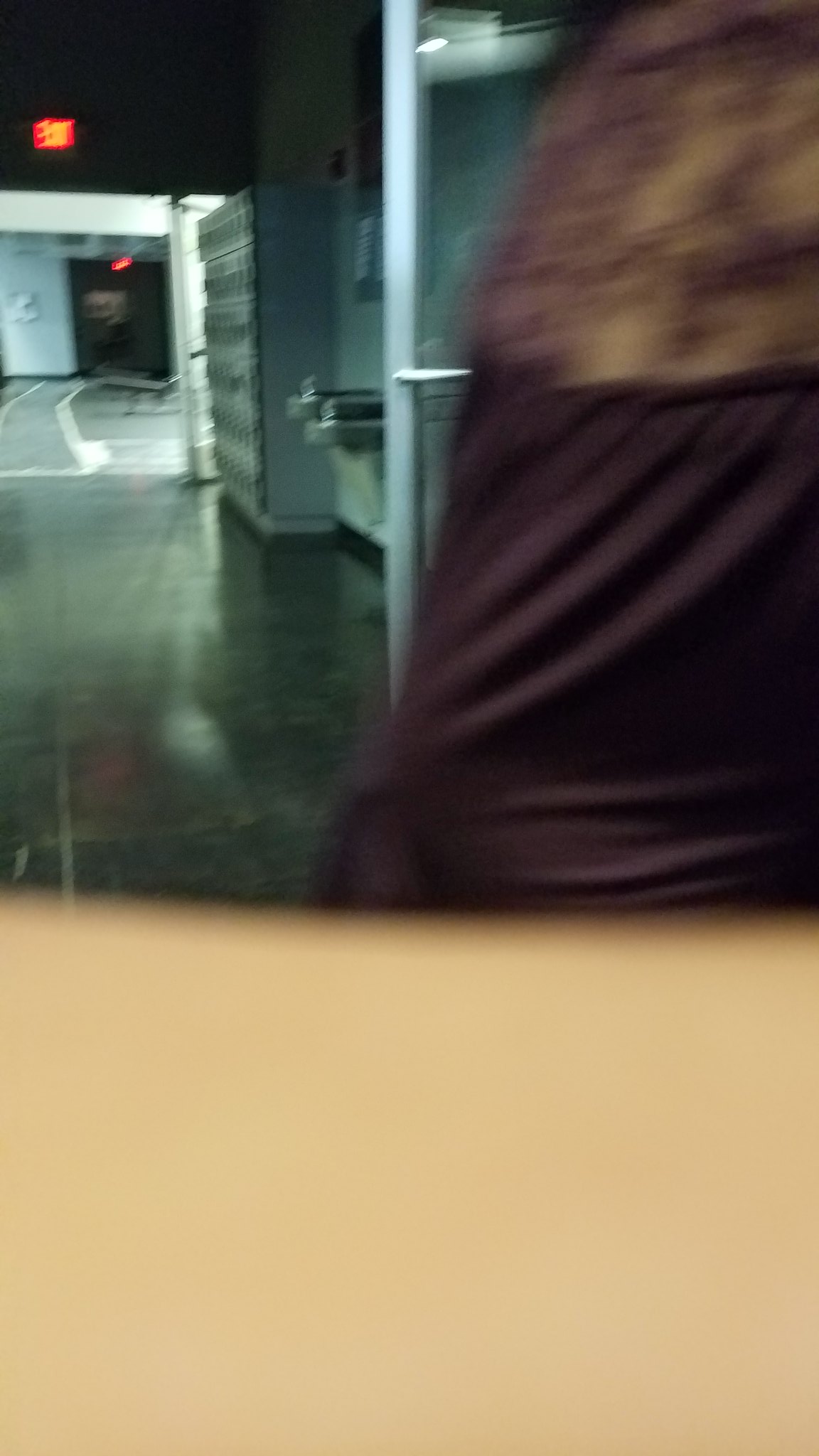This photograph captures an indoor hallway, potentially within an office building or school. The framing suggests it might be an accidental shot due to an obstruction partially covering the camera lens. On the right side of the hallway, two drinking fountains are visible, positioned beneath a cabinet or locker-like structure, hinting at the functional nature of the space. The image conveys a sense of utility and order, common in institutional or professional settings.